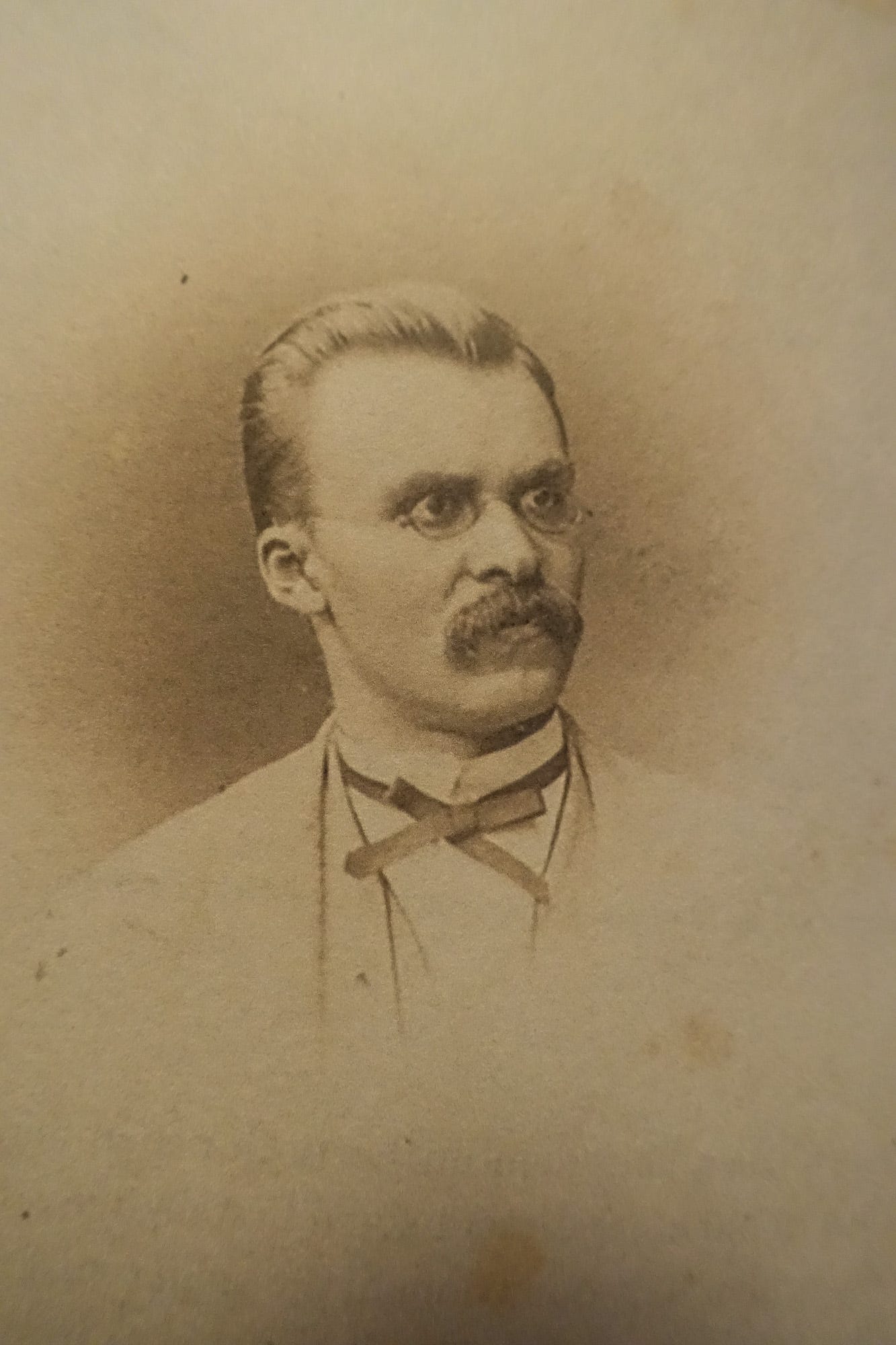The image is an aged sepia-toned drawing of a distinguished, middle-aged white male, who exudes an air of importance. The paper has browned with time, enhancing its vintage aesthetic. The man has a receding hairline with short, light-colored hair neatly slicked back. He sports a pair of small, circular wire-framed glasses and a prominent, walrus-like mustache, with no accompanying beard or goatee. His expression is stern and intent, with sharp, piercing eyes directed slightly to the right side of the image. His lips are parted just enough to reveal a hint of his teeth. He is dressed in a white shirt adorned with a thin, ribbon-style bowtie, complemented by a light-colored, open jacket. The edges of the image are somewhat blurry, drawing a stark contrast to the meticulously detailed depiction of his face.